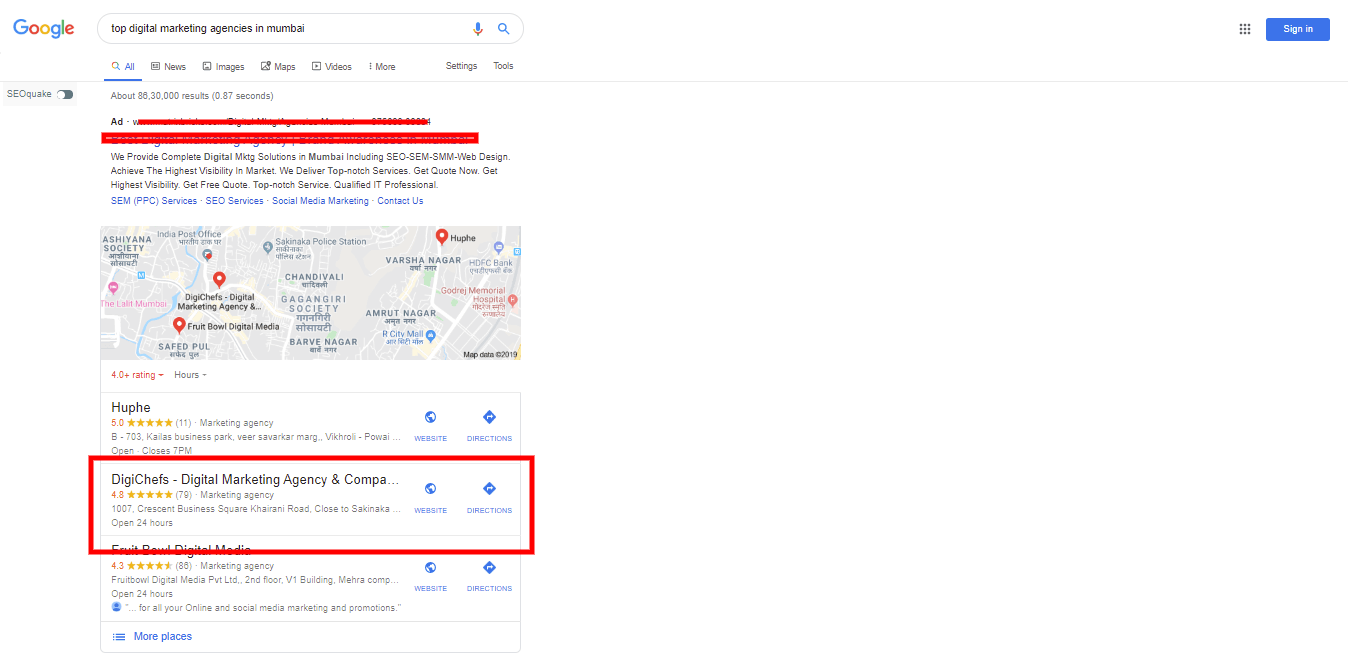The image displays a Google search results page for the query "top digital marketing agencies in Mumbai." The search engine results show various listings, with a particular ad crossed out in red marker. One highlighted result is for the DigiChefs Digital Marketing Agency, distinguished by a red rectangle. DigiChefs boasts 79 reviews and an impressive rating of 4.8 stars. The agency is located at 1007 Crescent Business Square on Kalyani Road, near Sakinaka. It is noted for being open 24 hours. To the right of this information are clickable blue icons for the website and directions. In the top right corner of the screen, there's a blue "Sign in" button followed by an icon consisting of nine dots. The area next to the search results is a blank white space.